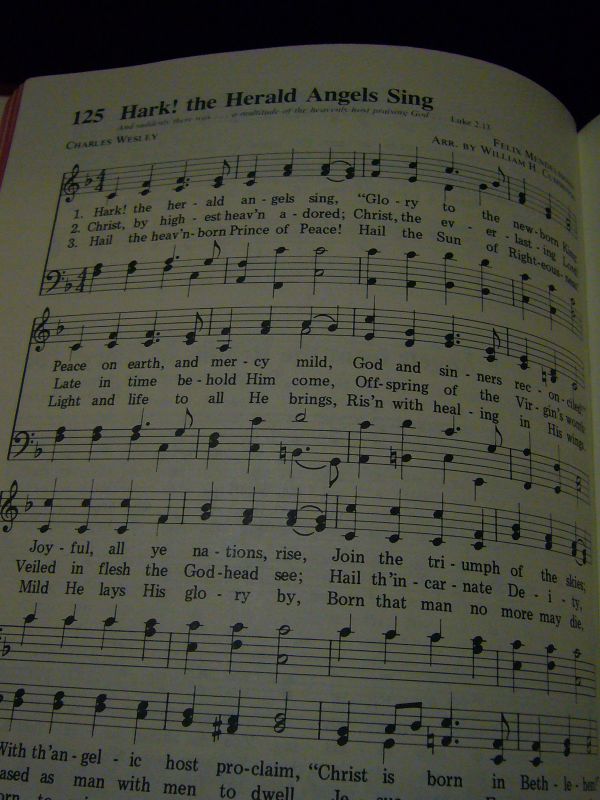This image is a close-up of the first page of a gospel sheet music book showing "Hark! The Herald Angels Sing" by Charles Wesley, labeled as Number 125. Below the title on the top left, "Luke 2.12" is inscribed, giving a scriptural reference for the hymn. The sheet music features three visible lines of staff notation with black musical notes detailed on five horizontal lines with four spaces in between, typical of traditional sheet music. The lyrics for the hymn are placed in between the treble and bass clefs. The bottom line of the sheet music is cut off in the image, along with the contents of the second page. This image captures the essence of a music book used for church performances or music classes, offering both musical notation and lyrical guidance for the song. The photograph itself is taken in such a way that parts of the page are missing, focusing closely on the main portion of the first page. The overall theme of the image is distinctly religious and instructional, showcasing a beloved hymn with historical and spiritual significance.